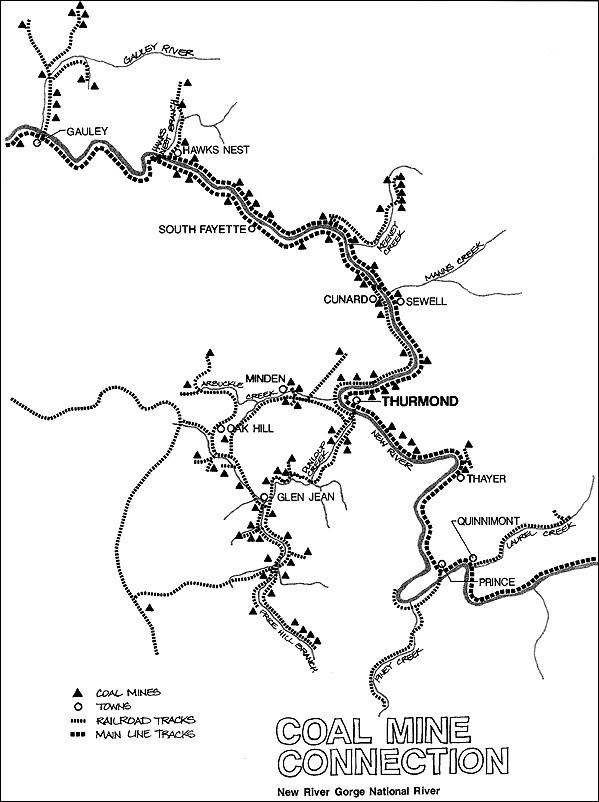The image is a meticulously detailed, black-and-white sketch of a coal mine network within the New River Gorge National River area. Dominating the vertical rectangular illustration, the central map highlights multiple coal mines, represented by solid black triangles, with labels such as Thurmond, Gully, Hawk's Nest, and others. Surrounding text elements, like "Coal Mine Connection" in bold, outlined letters and "New River Gorge National River" in slightly smaller, solid black text, clearly define the context of the map. A small, essential key in the bottom left corner uses black triangles to denote coal mines, open black circles for towns, thin dashed lines for railroad tracks, and thick dashed lines for mainline tracks. The meticulously drawn black ink lines on the white background give the map an aged, hand-drawn appearance. This visual guide intricately maps out how the coal mines are interconnected by a network of railroads and towns, all cohesively positioned to navigate the region’s rich industrial landscape.